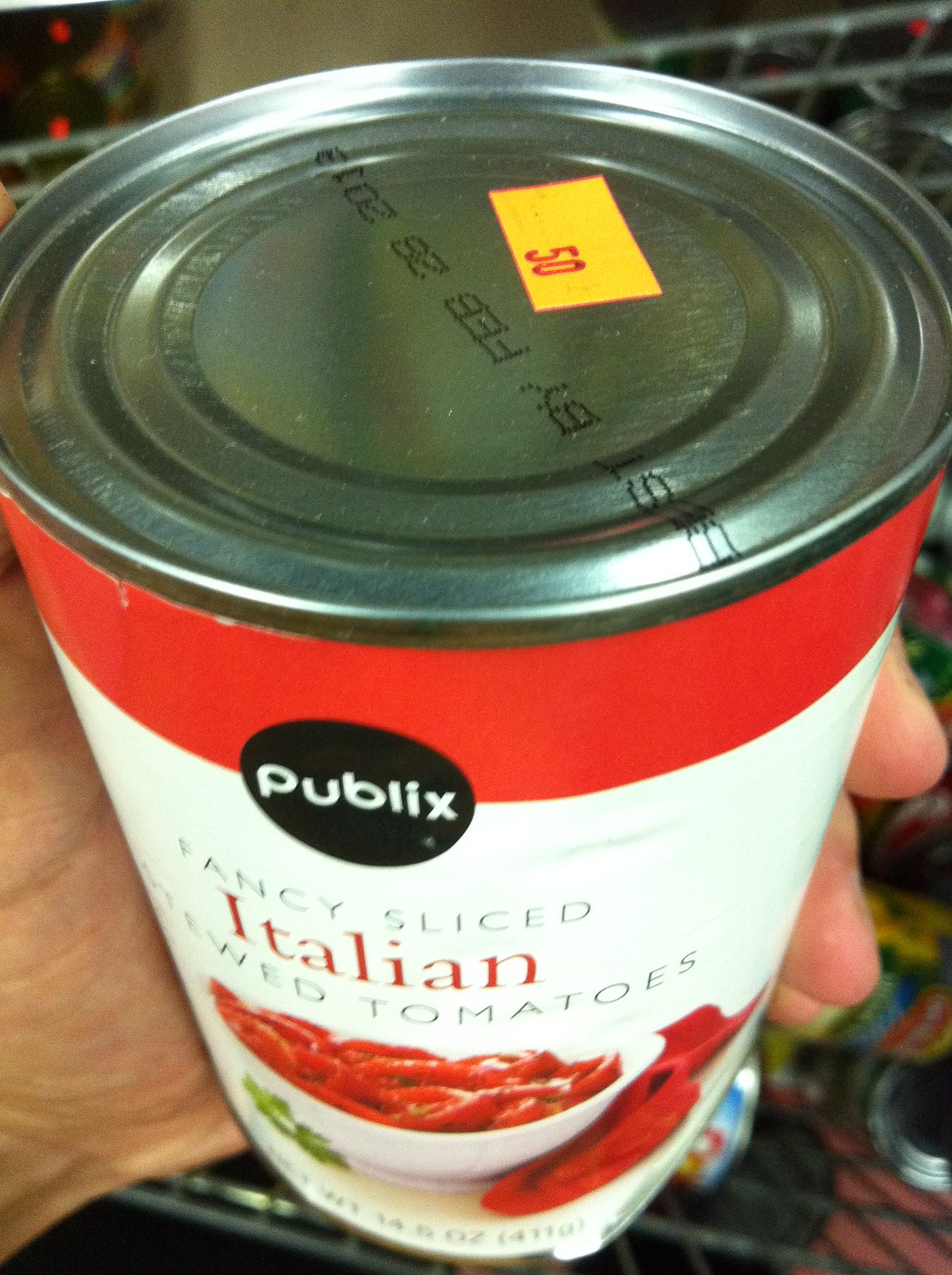In this photograph taken inside a grocery store, a person is holding up a 14-ounce can of Publix-brand Fancy Sliced Italian Stewed Tomatoes. The can features a predominantly white label with a red accent at the top, showcasing an appetizing image of a white bowl filled with the stewed tomatoes. Notably, the can has a "Best By" date stamped as February 28, 2013, and a discount sticker indicating a price of 50 cents. In the background, there is a partial view of a shopping cart situated in the middle of an aisle, subtly adding to the store atmosphere.